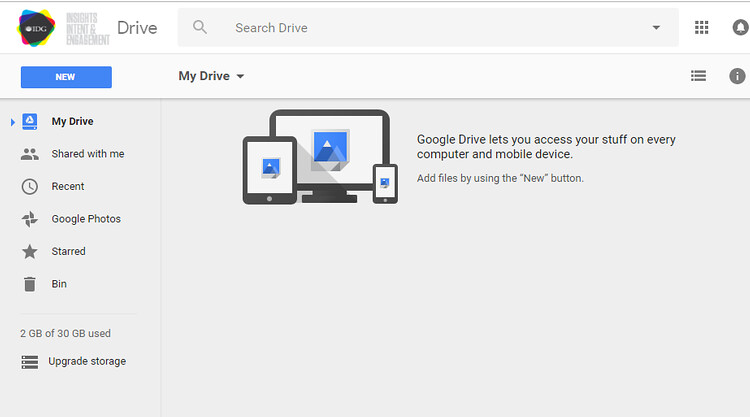The image is a detailed screenshot of a laptop screen displaying a Google Drive interface. The interface has a light pale gray background covering the top section, adorned with an indistinguishable logo. This logo comprises overlapping blue, yellow, and red triangles, with a black triangle in the middle featuring white lettering. Text within the logo appears to mention "Insights, Intent, and Engagement," followed by the word "Drive." 

Below the logo sits an elongated search bar labeled "Search Drive" accompanied by a magnifying glass icon on the right, and a down arrow for additional options. Adjacent to the search bar is a small menu icon depicted as three rows of three small squares, followed by a bell icon and a dark circle near the top right.

A secondary row beneath this section displays a blue rectangle with "New" in white lettering, and "My Drive" in tandem with a dropdown arrow. Additional icons include a menu icon and an information icon (a white "i" on a gray circle).

The main interface features a left-side navigation panel with several icons and text descriptions: 
- A folder icon labeled "My Drive"
- A people icon with "Shared with me"
- A clock icon labeled "Recent"
- A pinwheel icon with "Google Photos"
- A star labeled "Starred"
- A trash can icon with "Bin"

At the bottom of the navigation panel, it indicates the storage usage: "2 GB of 30 GB used," with an option labeled "Upgrade storage."

The central part of the screen showcases a graphical illustration of a computer monitor, tablet, and smartphone, all outlined in charcoal gray with white screens displaying a stylized snow-capped mountain peak. A text below the images reads, "Google Drive lets you access your stuff on every computer and mobile device. Add files by using the 'New' button."